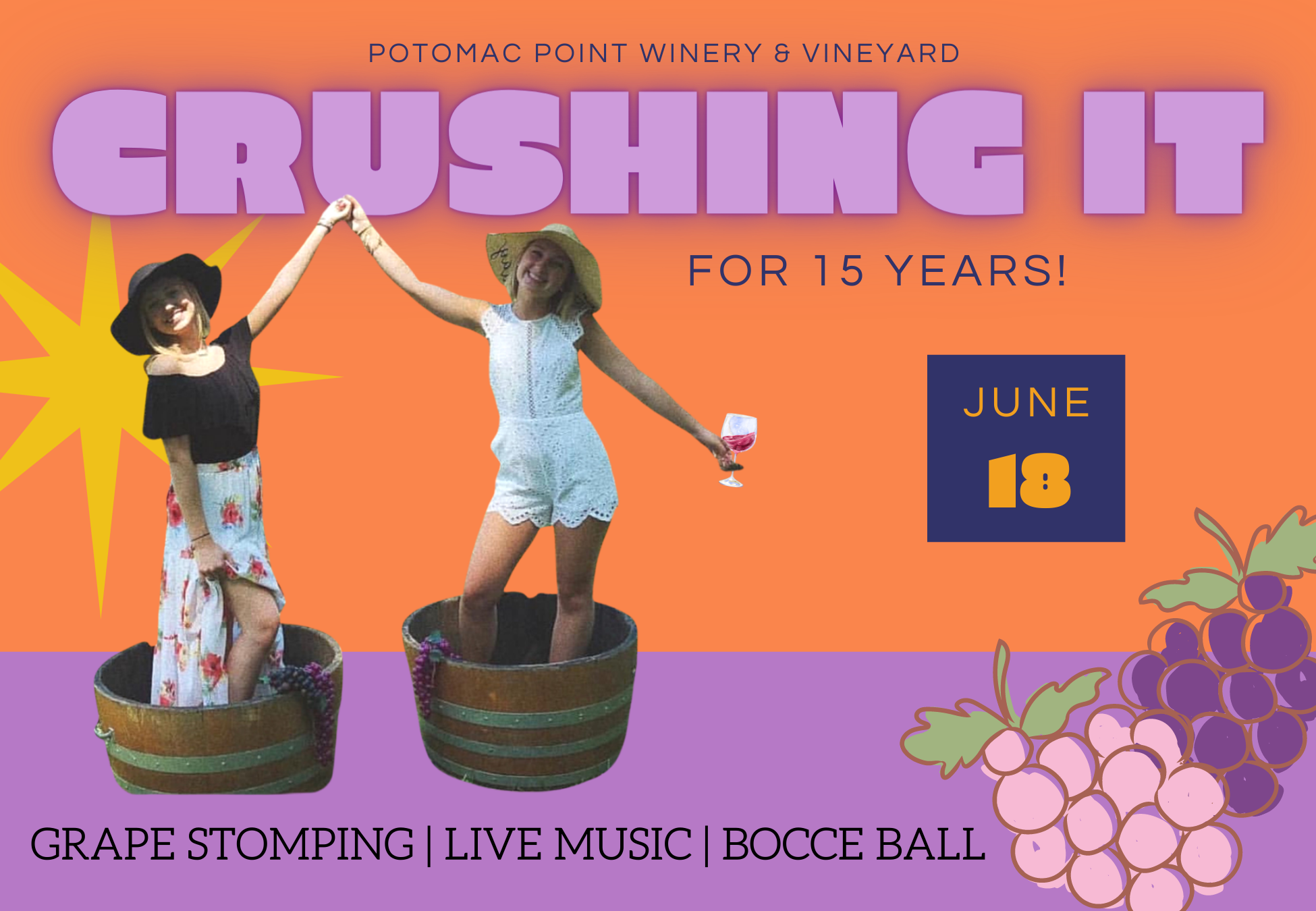This vibrant, full-color digital poster with no border is square-shaped and features an orange and purple background. At the top, in small all-caps text, it reads "Potomac Point Winery and Vineyard." Below that, in large, bold purple letters, it says "Crushing It for 15 Years." The event date, June 18th, is highlighted in a blue square with yellow text on the center left of the image, around a drawing of a stylized sun. 

The focal point showcases two young women standing in wooden barrels, enthusiastically stomping grapes. One woman, dressed in a white jumpsuit with shorts and wearing a sun hat, is holding a glass of wine. The other woman, wearing a black short-sleeved top and a skirt hitched up over her knee, also sports a sun hat. They are holding hands, emphasizing the joyous and communal spirit of the event.

In the lower right corner, there are two artistic renderings of grape clusters, reinforcing the grape-stomping theme. Across the bottom of the poster, the activities "Grape Stomping, Live Music, and Bocce Ball" are prominently listed, inviting viewers to join the celebration. This detailed and whimsical artwork captures the festive essence of Potomac Point Winery and Vineyard's 15th-anniversary event.